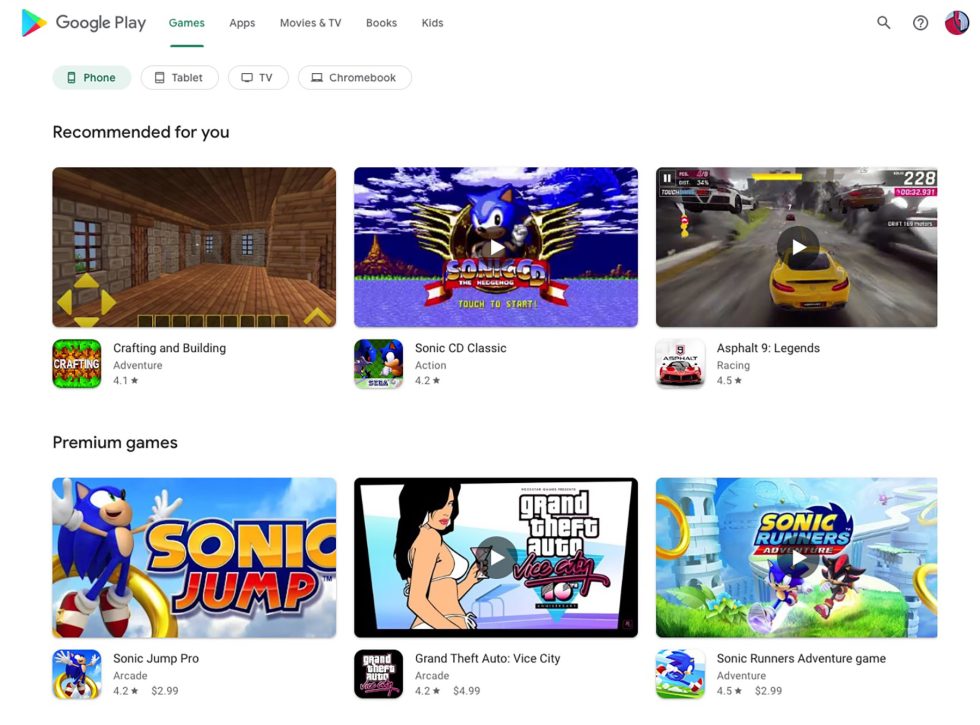This image captures the home screen of the Google Play Store app, specifically showcasing the Games tab. At the top of the screen, the iconic Google Play logo is displayed alongside the multi-colored Play button. Below the logo, several categories are arranged in tabs: Games, Apps, Movies & TV, Books, and Kids. The user is currently viewing the Games tab.

Further down, a device filter option is available, allowing the user to select between Phone, Tablet, TV, and Chromebook, with the Phone tab actively selected. Below the filter, a series of curated game lists is presented.

The first list, titled "Recommended for You," features the following vertical arrangements:
1. **Crafting and Building** - Categorized under Adventure, this game holds a 4.1-star rating. The thumbnail features a scene reminiscent of Minecraft, showcasing a wooden house.
2. **Sonic CD Classic** - An Action game with a 4.2-star rating. The thumbnail displays Sonic the Hedgehog striking his signature pose against a backdrop of ocean scenery with mountains and sky.
3. **Asphalt 9: Legends** - A Racing game rated at 4.5 stars. The thumbnail portrays a car in the midst of a high-speed race.

Below the "Recommended for You" section, another list titled "Premium Games" includes:
1. **Sonic Jump Pro** - An Arcade game with a 4.2-star rating, priced at $2.99.
2. **Grand Theft Auto: Vice City** - Also categorized under Arcade, this game has a 4.2-star rating and is priced at $4.99.
3. **Sonic Runners Adventure Game** - An Adventure game with a 4.5-star rating and a price of $2.99.

Each game listing is accompanied by a representative thumbnail and star rating, providing a snapshot of the game's visuals and community ratings.